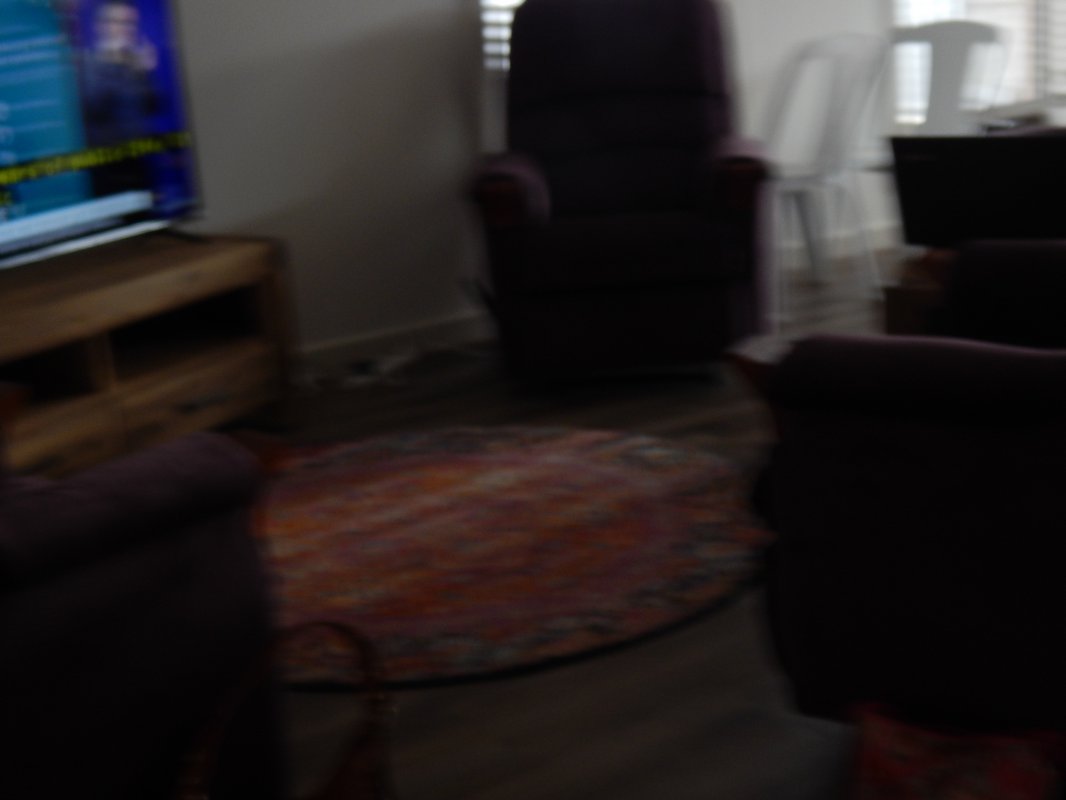This image, which is somewhat square in shape, is characterized by noticeable blurriness, lacking any clear focal points. Despite the lack of clarity, the setting appears to be the interior of a house, possibly a living room. Within the image, a brown TV stand is visible, hosting a flat screen television that is turned on. Surrounding the TV stand are several pieces of seating furniture, which seem to be darker maroon in color, possibly including three different chairs or couches. A circular rug with shades of red, orange, and brown is centrally placed on what appears to be a brown floor. Through the blur, another room is faintly discernible, featuring white, possibly plastic, outdoor-style chairs and what might be an additional table.